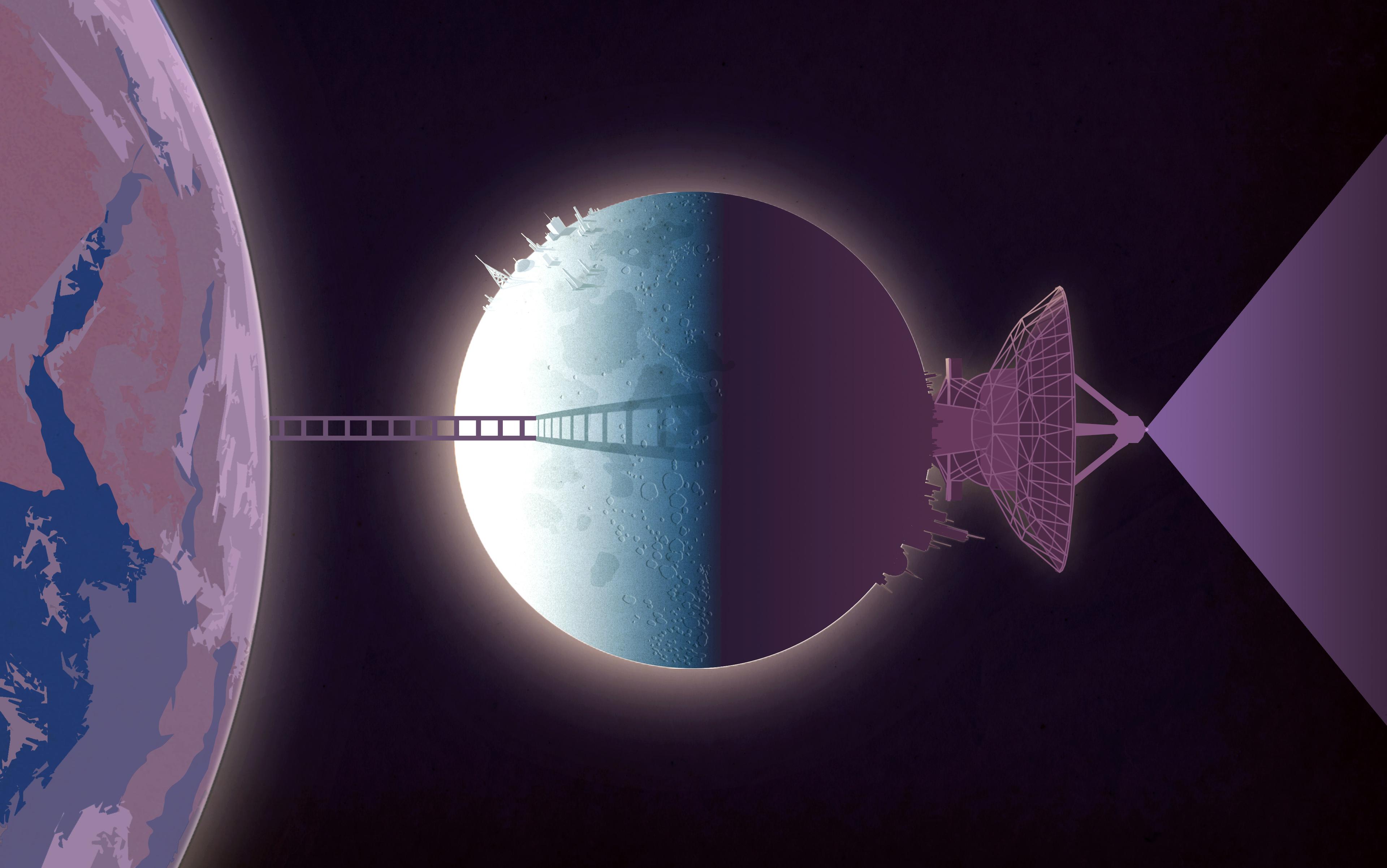The image depicts a surreal scene of a ladder extending from the Earth, which peeks partially into frame from the left, to the moon at the center. The Earth showcases some discernible continents, clouds, and ocean in an array of blue tones. The moon, illuminated on its left side, reveals a collection of buildings suggesting a small civilization. Dominating the right-hand side of the moon, which is cloaked in shadow, is a large satellite dish. This satellite emits a striking cone of purple light that extends outward into the dark expanse of space. The ladder, seemingly defying physics, bridges Earth and moon, casting a shadow across the lunar surface. The rest of the image is enveloped by the blackness of space, emphasizing the celestial and fantastical elements of this cosmic connection.